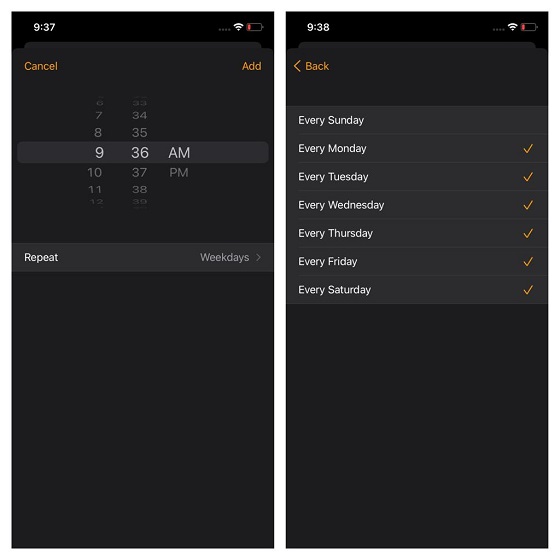The image comprises two side-by-side screenshots of an Apple iPhone's Clock app in dark mode, showcasing an older interface design. 

On the left screenshot, the user is in the process of setting an alarm for 9:36 AM. The interface is simplistic and features minimalist design elements. At the top, prominently displayed in dark yellow font, are the options to 'Cancel' or 'Add' the alarm. Below the alarm time setting, there's a 'Repeat' option, which the user has configured to activate on weekdays. 

The right screenshot delves deeper into the repetition settings, displaying a menu where the user can choose specific days for the alarm to go off. Here, seven options are listed: every Sunday through to every Saturday. The user has selected all days except for Sunday, marked by yellow checkmarks beside Monday through Saturday. At the top-left corner of this menu, a 'Back' button is visible, allowing the user to return to the previous screen.

The entire interface is set in a dark gray, indicative of either the dark mode or the standard theme for this version of the Clock app.